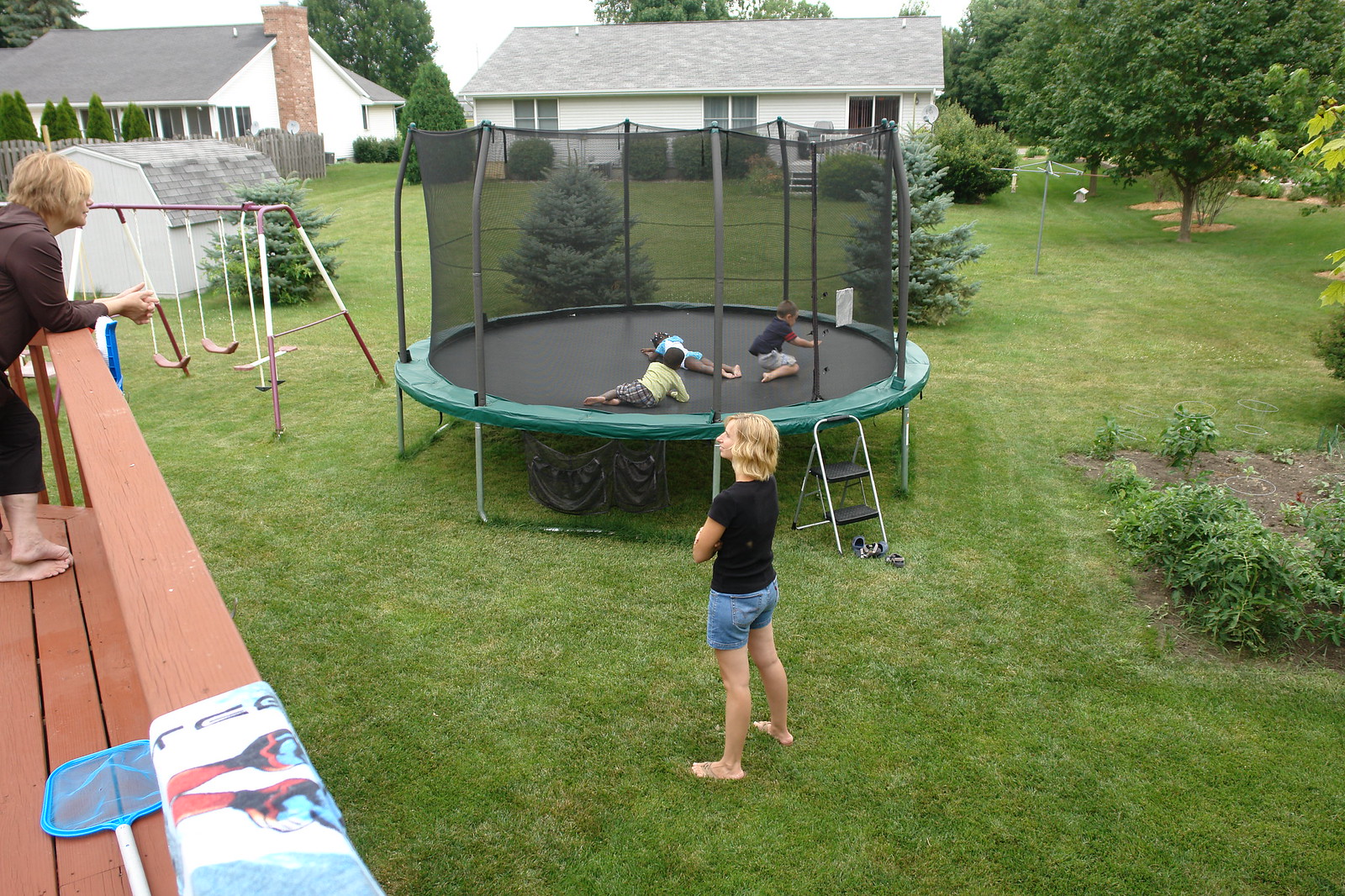The photo showcases a vibrant backyard scene during summertime. At the forefront stands a mom, barefoot on the lush green grass, wearing denim shorts and a black t-shirt, with her blonde hair catching the light. She is engaged in conversation with an older woman, likely the grandmother, who is barefoot and dressed in a black sweatshirt and three-quarter length pants. The grandmother leans over the wooden red-stained deck's rail, her blondish hair slightly tousled. A mesh pool net and a beach towel are also visible on the deck.

The spacious and well-maintained yard features a green trampoline with protective netting. Three children are playing on it: two are lying down while one is kneeling. Nearby, a classic metal swing set with a teeter-totter and sling-style swings stands alongside a small barn-shaped shed. 

The background reveals a seamless expanse of the green lawn leading into the neighboring yards, punctuated by tall spruce and pine trees. A vegetable garden, possibly with tomato plants, is situated to the right. The outdoor space is accentuated by small details like bird feeders and diverse flora, adding to the idyllic backyard scene. Two white ranch-style houses are partially visible beyond a mix of open space and a privacy fence adorned with Leland cypress or cedar trees, underlining the serene, communal atmosphere.